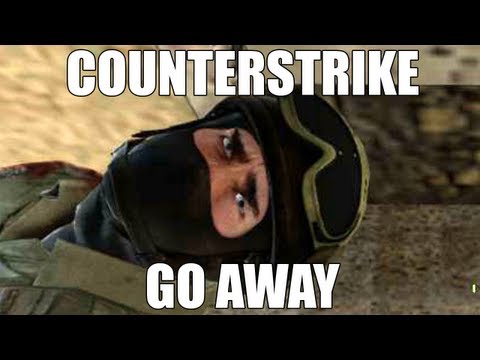The image appears to be computer-generated and features a soldier lying horizontally, with only his head and the upper part of his body visible. The background includes a black strip at both the top and bottom of the image. At the top, in all-capitalized white letters, is the word "COUNTER-STRIKE," and at the bottom, similarly capitalized, is "GO AWAY." The soldier wears a black mask that covers his entire forehead, mouth, and sides of his face, but leaves his intense blue eyes and thick, dark eyebrows visible. He has a pair of goggles resting on the top of his head. The soldier appears to be wearing military attire, including a green collared shirt or khaki coat and possibly a camo vest. The background suggests he is either on concrete or in a desert-like environment, with hints of sand visible to his left. He has an intense expression on his face, and the image suggests a wartime setting.